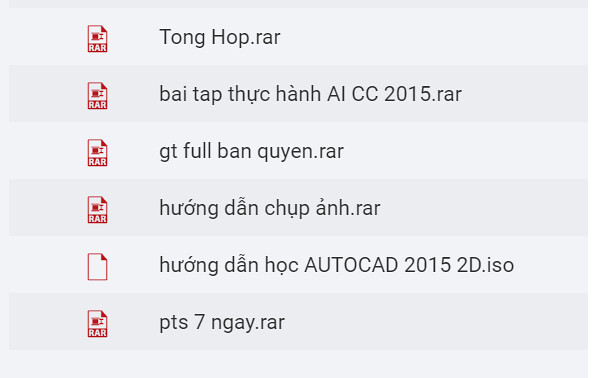The image depicts a dark gray to light gray gradient background divided into six horizontal bands, each containing a file icon and its corresponding file name. The icons are primarily standard file icons featuring a white piece of paper with the top right corner folded over. Each icon has a small red square with the letters "RAR" in white, except for the fifth one which is just a blank piece of paper with the folded corner and a red outline.

From top to bottom:
1. A file icon with "RAR" inside a red square labeled "tonghop.rar".
2. A similar icon labeled "baytapthukhanaicc2015.rar" in an Eastern or Southwestern Asian script.
3. The same icon labeled "gtfulfanhuyen.rar" in another language.
4. The same icon labeled "huangdanchuan.rar" in a similar script.
5. A different icon, just a red-outlined paper with a folded corner and no "RAR", labeled "huangdanhokautocad20152d.iso".
6. The standard icon again labeled "pts7ngay.rar".

The repetitive visual elements combined with minor variations in iconography effectively illustrate the nature of the files in the screenshot.